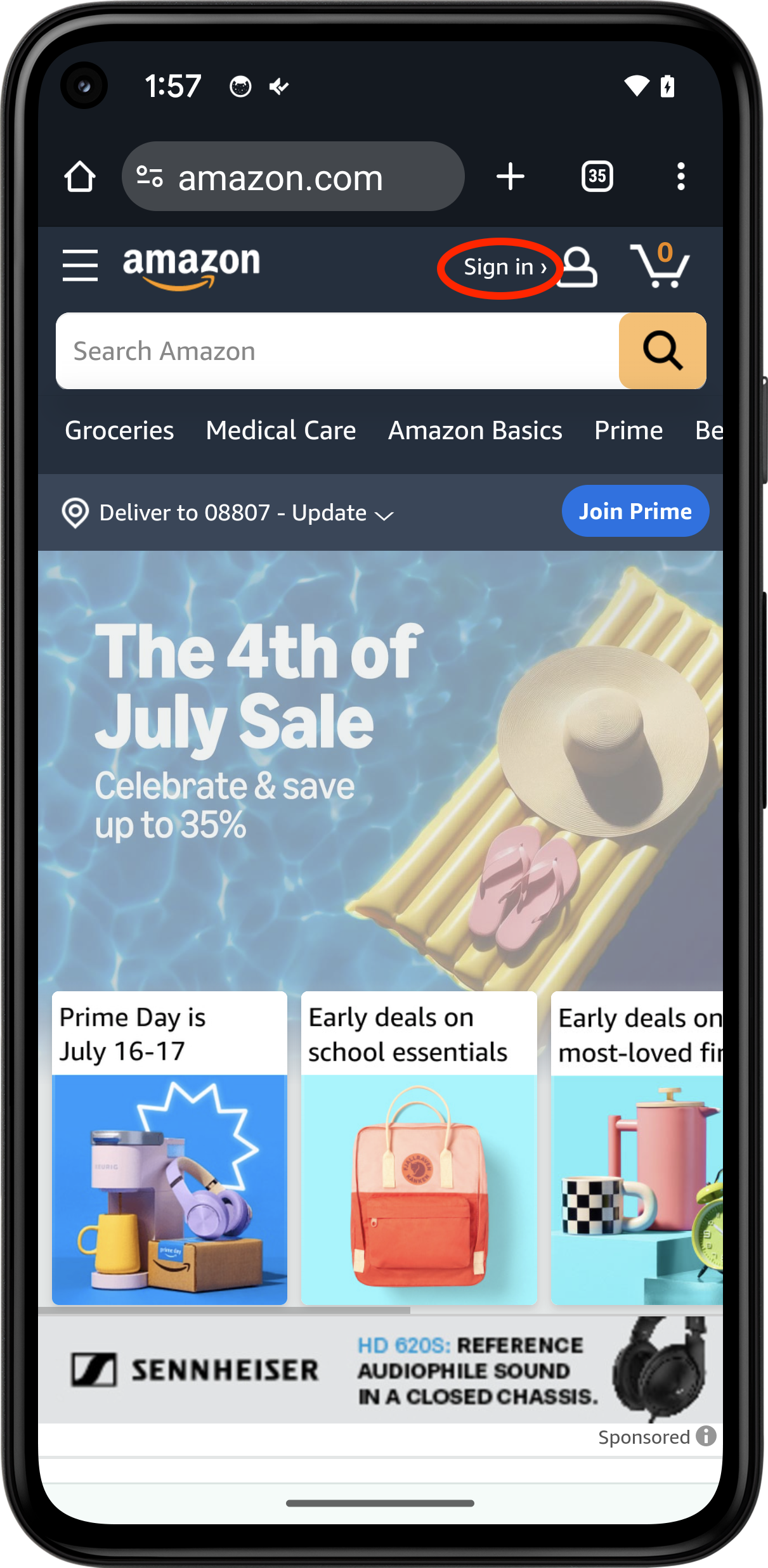This image depicts a screenshot from a mobile phone displaying the homepage of Amazon.com. The URL at the top confirms the website. Notably, the "Sign-In" button is prominently circled in red, which is an unusual feature for the standard browsing experience on Amazon's mobile site, indicating it is likely an annotation intended for instructional purposes, perhaps to guide users on accessing their accounts.

The page itself is replete with Amazon's typical features. At the bottom, visible sections showcase several popular deals, including a digital photo frame and a Nerf gun, highlighting the variety of discounted products available. Central to the page is a large banner announcing "Cyber Monday," encouraging users to "shop new deals all day." This suggests the screenshot was taken during the Cyber Monday sales event, typically occurring in late November following Black Friday.

Additionally, a secondary banner promotes "Alex Rider," an IMDb TV original series, with an invite to watch it for free. These banners and product highlights capture the essence of Amazon's dynamic homepage during a major annual sales event.